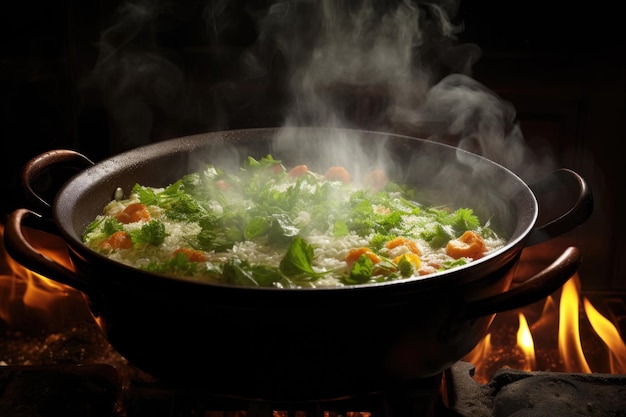The image is a professional photograph of a large, black, stone or cast iron pot with four handles, two on each side, against a very dark background. The pot is placed on an open stove with stones and is surrounded by visible flames at the bottom, indicating intense cooking activity. Inside the pot, which is either boiling soup or a stir-fry, there is steam rising prominently, reinforcing the sense of heat and active cooking. The contents include white rice, fresh broccoli, parsley, carrots, something orange like bell peppers, and possibly noodles or meat. The picture, which is slightly elongated to accommodate the large pot, captures the essence of a hot, steaming dish in a rustic and intense culinary setting.